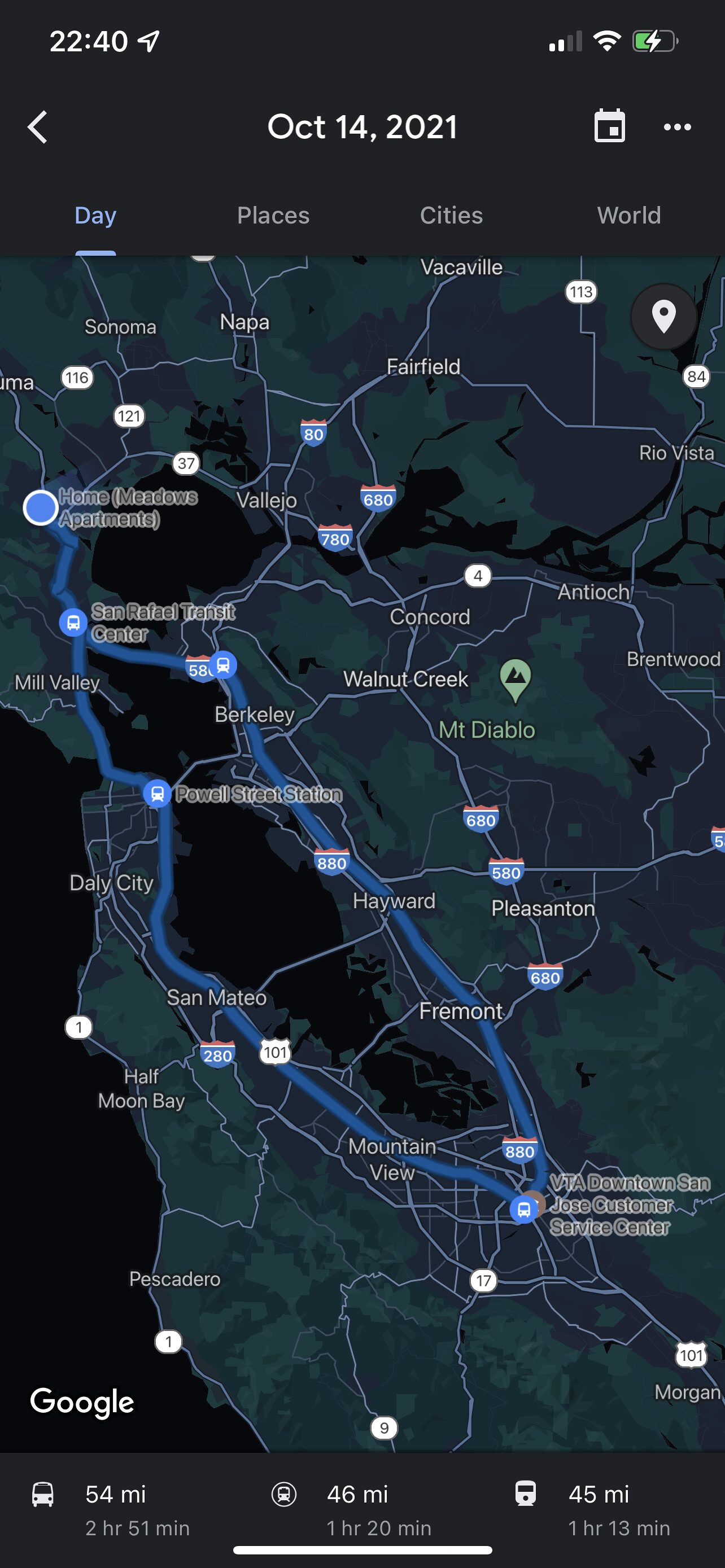This photo showcases a detailed map of California, highlighting various cities such as Berkeley, Concord, Walnut, Mount Diablo, Pleasanton, Fremont, Half Moon Bay, San Mateo, and Mountain View. A distinct blue-outlined circle encompasses a central area on the map. At the bottom of the image, there's a timeline bar displaying various travel durations: 54 minutes, 2 hours and 51 minutes, 46 minutes, 1 hour and 20 minutes, 45 minutes, and 1 hour and 13 minutes. Each time duration is associated with different modes of transportation, represented by symbols such as a car, metro, and trolley. Above this bar, the Google logo is prominently featured.